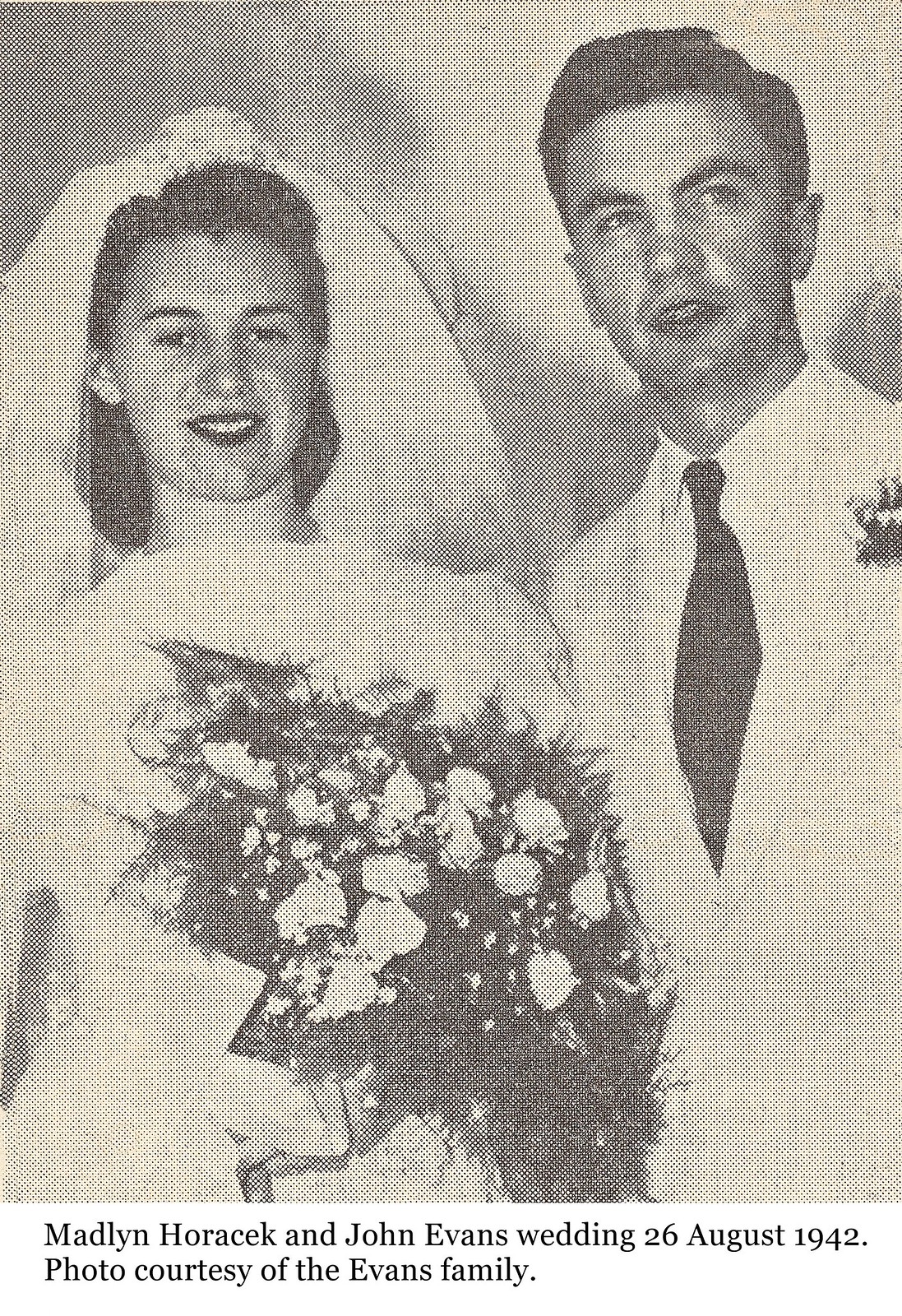A black and white photograph, grainy like an old newspaper clipping, captures the youthful bride and groom on their wedding day, 26 August 1942. The picture is courtesy of the Evans family, as indicated by the text beneath it. The groom, identified as John Evans, stands on the right. He has brown hair and wears a white suit with a black tie and a flower in his lapel, his gaze directed slightly above the camera. The bride, Madeline Horacek, stands beside him, wearing a white dress and veil that is pulled back over her hair. Her lips are adorned with lipstick, and she holds a bouquet that includes some evergreen leaves and white flowers, though their exact colors aren't discernible in the monochromatic image. Her direct gaze meets the camera, capturing the timeless moment of their wedding announcement.